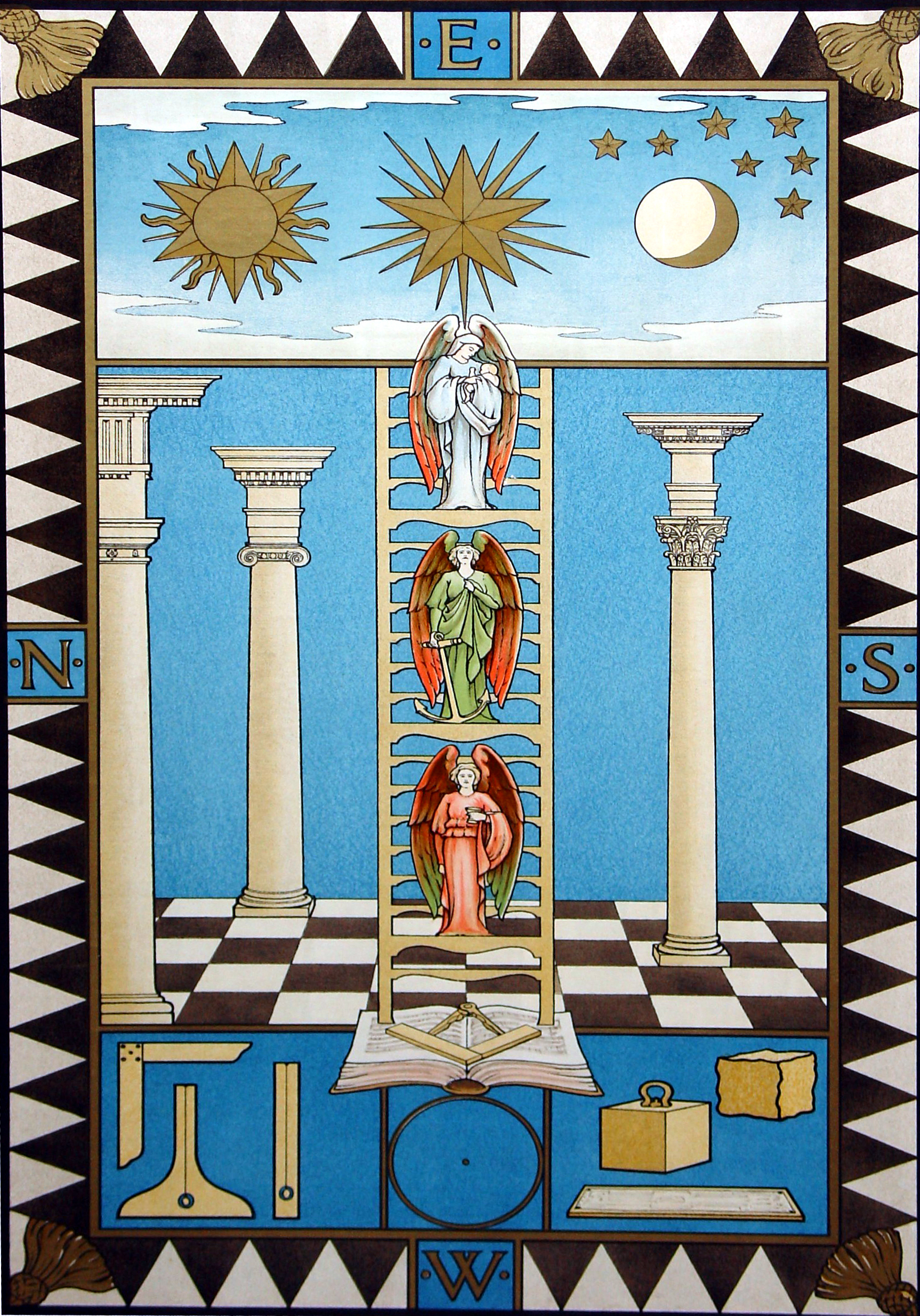The artwork is a vertically rectangular poster adorned with a faint brown border, encapsulated by an alternating black and white triangular pattern. Tassel-like brown shells with fringes embellish each corner of the frame, slightly distorting the triangle shapes. Surrounding the main image, directional letters—N, S, E, W—are placed in unconventional positions: north on the left and east at the top.

In the upper portion of the artwork, abstract illustrations depict the sun, moon, and stars nestled amidst clouds. The center features a grand gold throne set on a white and black checkered floor, flanked by three brown columns. Perched on the throne or a trellis ladder growing out of a book, three angels—or possibly religious figures—are positioned at different levels, one holding a baby, another bearing an anchor, and the third with a cup.

The lower section of the piece showcases various symbols and wooden tools, including what appear to be cubes with handles and measuring devices, amplifying the complexity and potential hidden meanings of the entire composition.